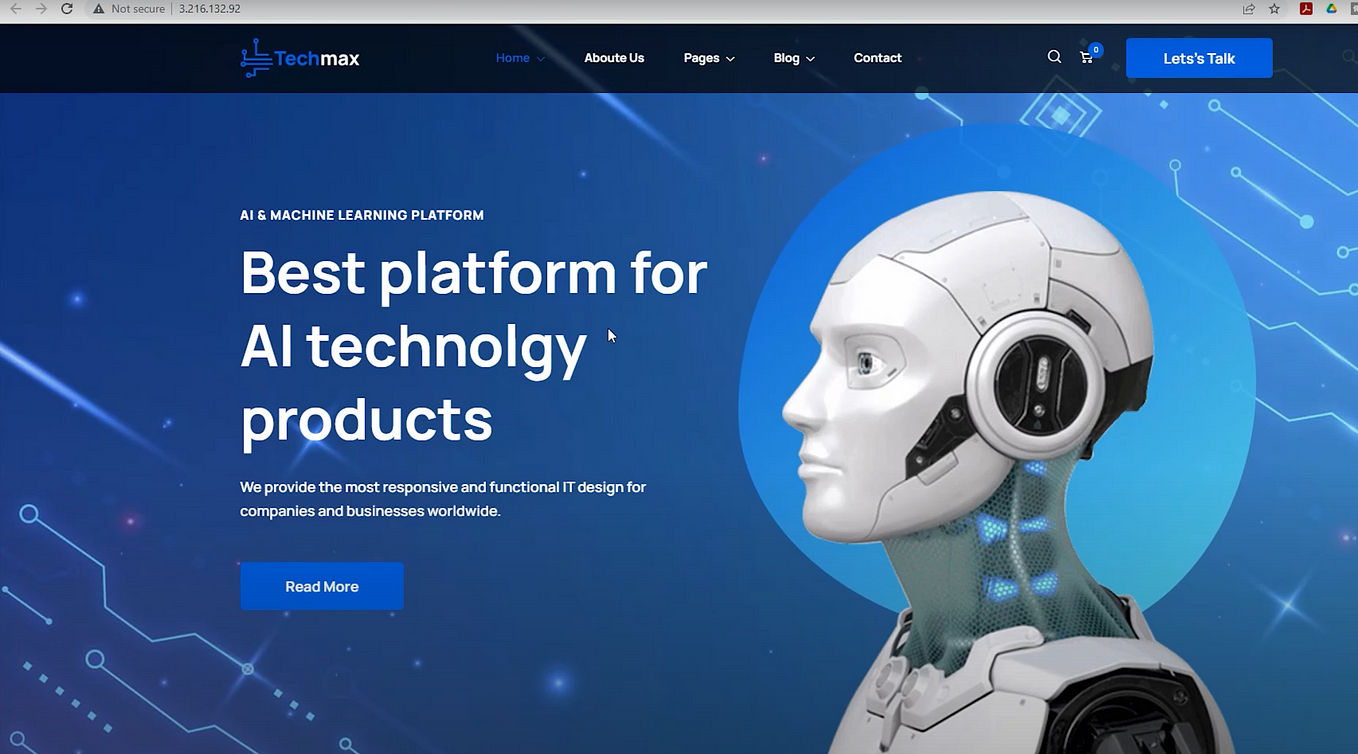The image features a computer screen displaying a website identified as "Tech Max." At the very top, the address bar indicates "Not Secure 3.216.132.92," accompanied by the usual browser symbols. Below this address bar is a thinner blue navigation bar featuring a series of clickable options in the center: “Home” in blue, followed by “About Us,” “Pages,” “Blog,” and “Contact” in white. To the far right of this navigation bar are a shopping cart icon and a blue rectangular button labeled "Let's Talk" in white.

The bulk of the webpage has a blue, digitally themed background with intricate patterns in the corners, giving it a spacey, tech-oriented feel. Dominating the right side of the page is an image of a robotic man, shown from the chest up and facing left. The robot has a white head, realistic eye, and appears to be constructed mostly of white robotic parts. A light blue circle frames the robot's head in the background.

On the left side of this robot image, small white text at the top reads “AI and Machine Learning Platform.” Below this, in larger white letters, is the slogan, “Best Platform for AI Technology Products.” Further down, in smaller white text, the site promises, “We provide the most responsive and functional IT design for companies and businesses worldwide.” At the bottom is a blue rectangular button with the words “Read More” in white text.